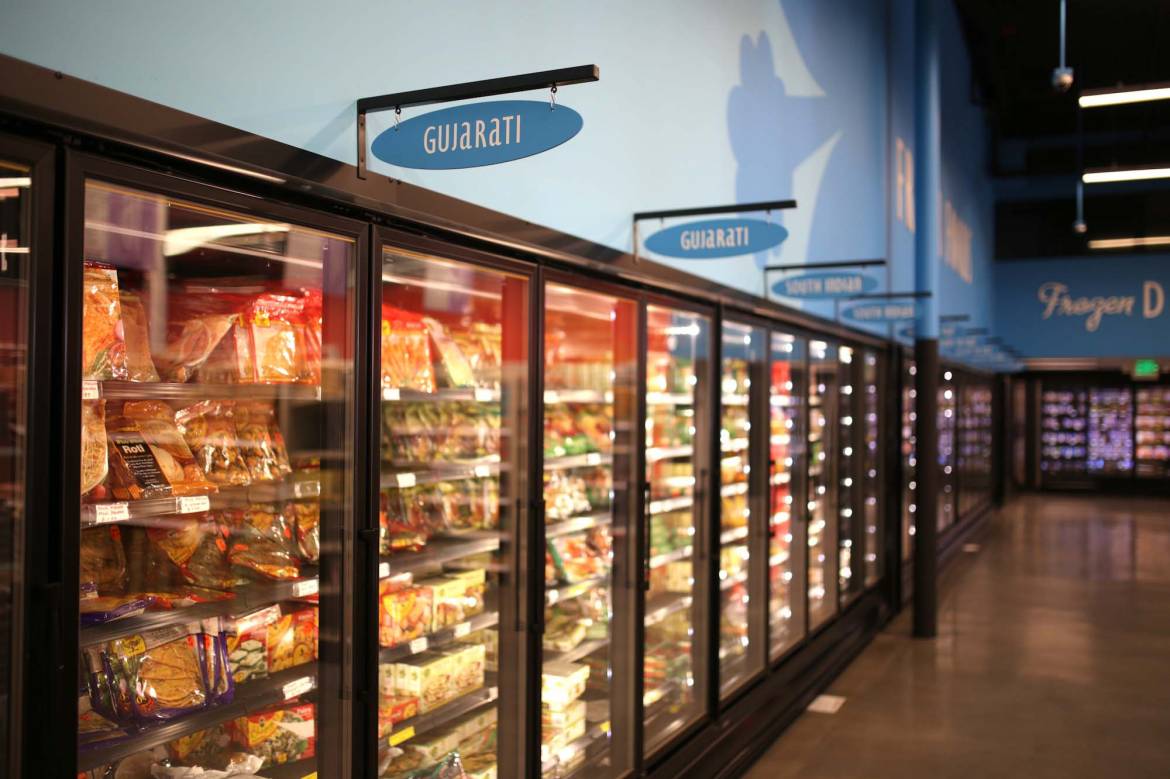In the image, the top wall features a gradient from an off-blue shade to a darker blue hue as it extends down the aisle, leading towards white lettering on the ceiling. Black hooks adorned with blue circles and white letters spell out "GUJARATI." The aisle is flanked by glass doors that reveal a variety of meats and frozen products. The dark gray floor contrasts with the black and blue pole in the distance. Overhead, white track lighting illuminates the scene, with a black ceiling adding to the visual depth. The glass doors have black handles and provide access to the refrigerated section. Within this section, the shelves are dark gray and lined with white stickers displaying the prices of the items for sale.